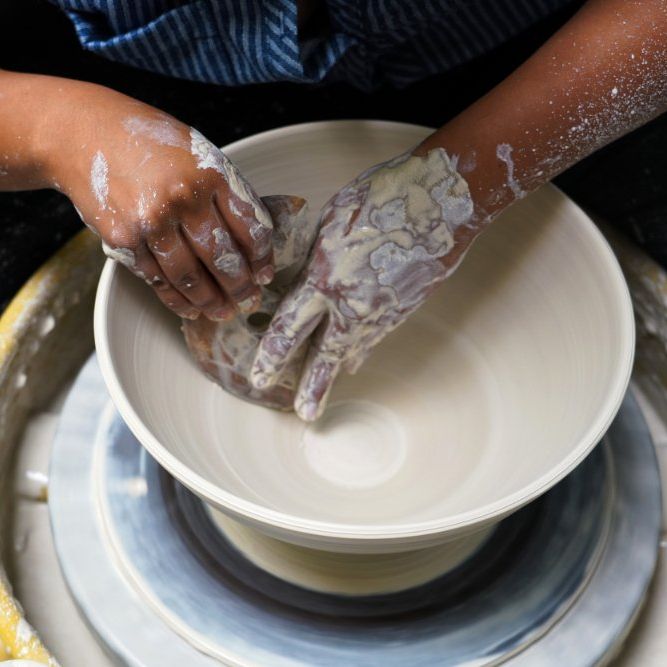The image captures a close-up, overhead view of a pottery wheel in motion, showcasing a bowl being meticulously crafted from light tan clay. The artisan, a woman with dark skin, is deeply immersed in her work, her hands and arms coated in both wet and dry clay. The wet clay presents a light tan hue, while the dried clay appears almost milky white. Her left hand, heavily laden with clay, shapes the exterior of the bowl, while her right hand, equipped with a small, indistinct tool, smooths the inside. The pottery wheel beneath her, partly visible, is silver with a blue spinning platform, and is partially outlined by a yellow band that holds the clay in place. The woman’s shirt, visible at the edge of the frame, features light and dark blue stripes. The square photograph, approximately five inches by five inches, captures the artistry and messiness of the pottery-making process.